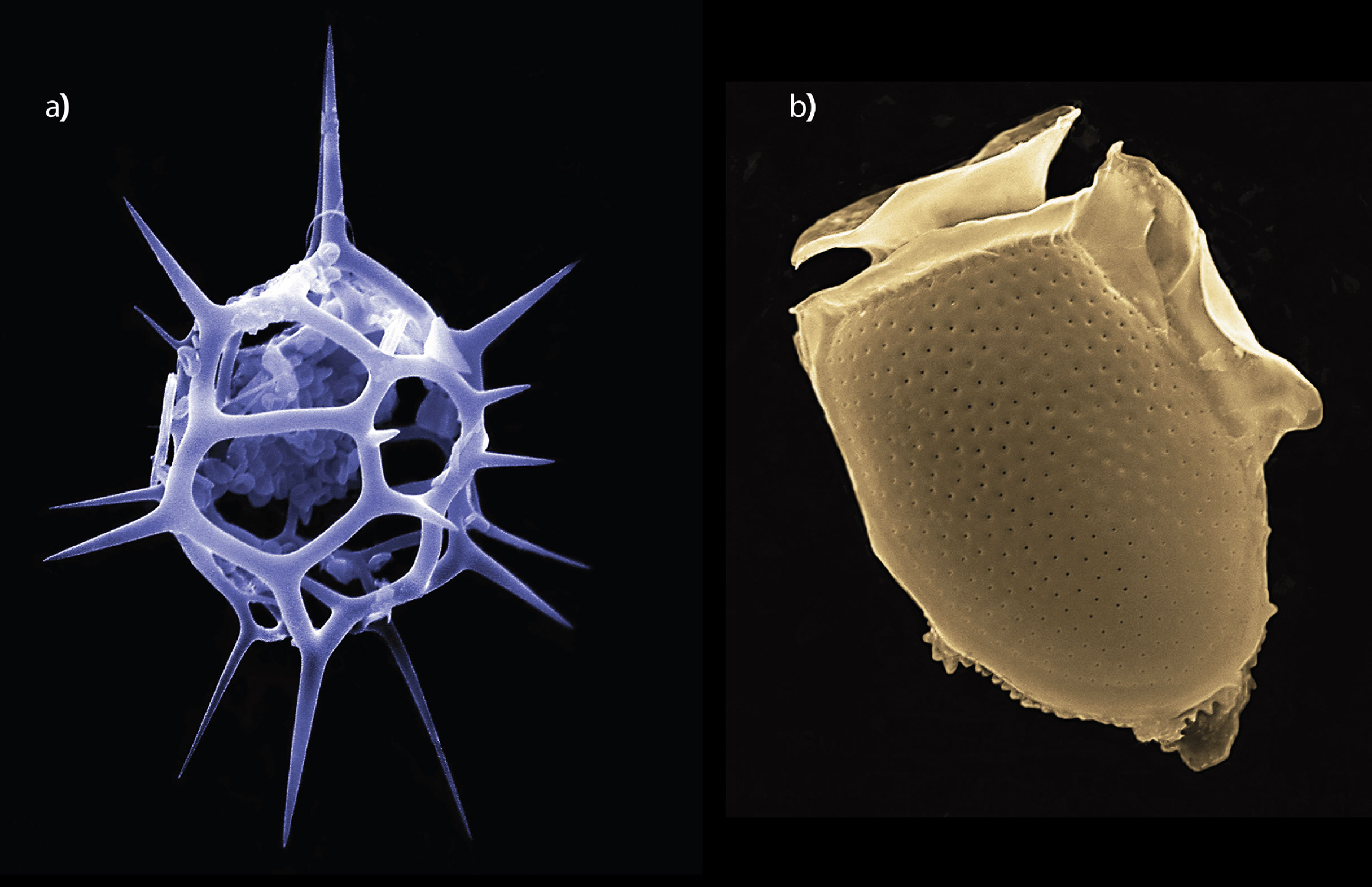Photograph against a completely black background featuring two numbered images, labeled A and B. 

Image A showcases a light purple spherical structure with numerous holes. Connected to the sphere are light purple rods, with several pointy light purple spikes protruding from the surface.

Image B has an oven mitt-like shape in a pale yellow hue. The body of the mitt features small dots, while flaps resembling wings extend from its bottom and right side.

Each element within these images is distinctly detailed against the stark black backdrop, emphasizing their unique shapes and colors.